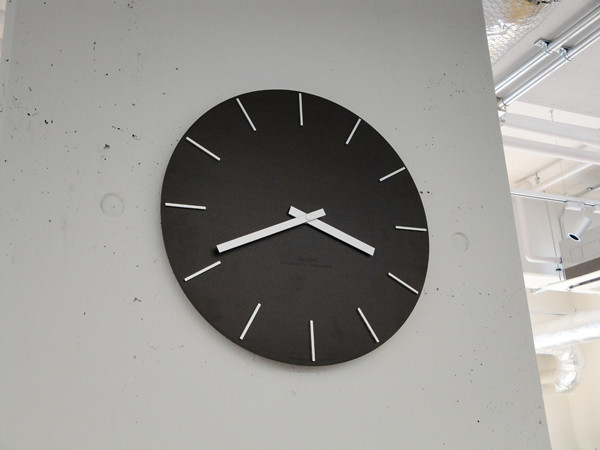This image depicts a large, ultra-modern black wall clock mounted on an off-white, industrial-style wall with visible imperfections, including small holes and smudges. The clock has a sleek, minimalist design with twelve silvery white dash marks indicating the hours, but no numbers or Roman numerals. Its silvery white hands show the time as approximately 3:41. The wall is part of an industrial building featuring a gray ceiling adorned with exposed metal piping, white track lighting, and assorted conduits that enhance the raw, unfinished look. The scene includes various industrial elements such as air conditioning units, light fixtures, and cords visible against the ceiling, contributing to the overall modern, industrial aesthetic.